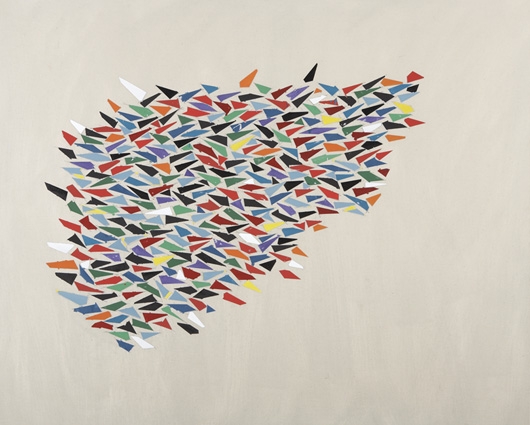This abstract artwork features a vibrant and complex arrangement of small, mosaic-like squares and various geometric shapes, predominantly triangles. The shapes are colorful, encompassing a wide spectrum including shades of red, orange, yellow, green, blue, light blue, black, gray, and dark shades of purple and dark red. These elements come together to form an irregular, oblong shape that could be likened to an arrowhead or the human liver, oriented with the upper part pointing to the right. The composition appears textured and possibly three-dimensional, though it is unclear whether it consists of paint, glass, or paper. The artwork rests on a gradient background of gray and white, while placed on a light tan surface, creating a striking contrast. This dynamic piece, central and leaning slightly to the left, captures the essence of abstract art with its pointy, jagged, and layered forms, offering a rich visual experience without the need for accompanying text.